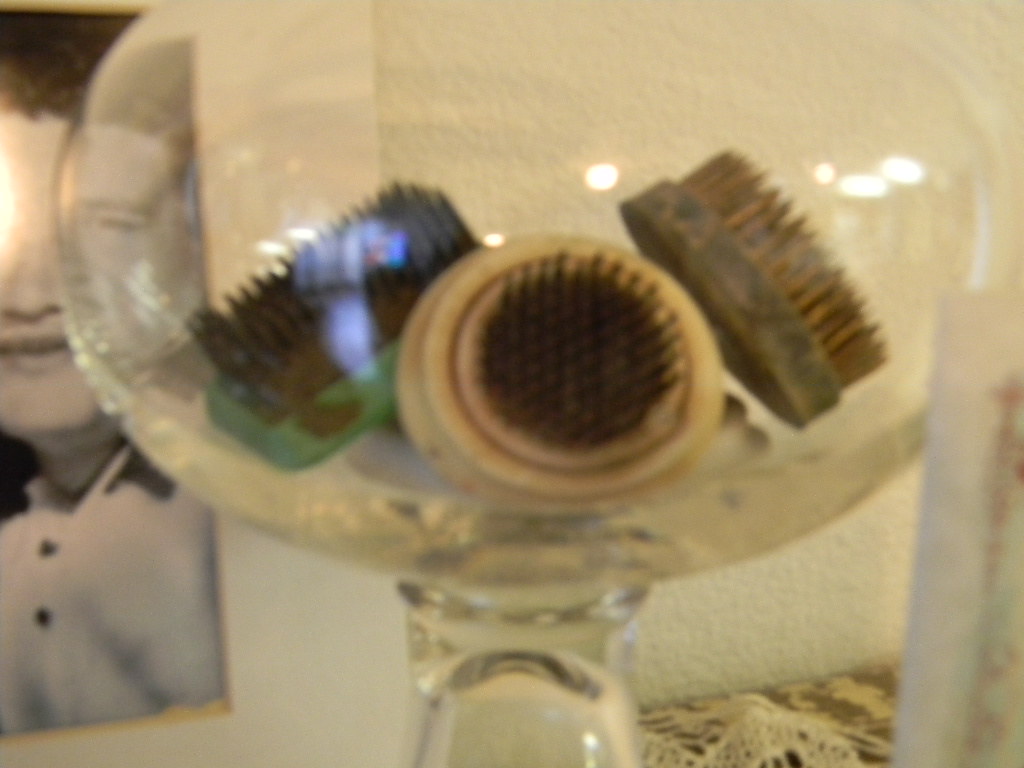The image features a close-up of a glass goblet with a pedestal base, containing three distinct scrub brushes. The brushes are used for scrubbing tasks, possibly for floors or dish pans. Two of them have round shapes, while the third one is rectangular with a green base. The round brushes have brown bristles, with one showing a cream-colored base and the other appearing to have a wooden handle with darker beige bristles. The bristles of all the brushes extend outward slightly less than their plastic or wooden holders, which allows for a firm grip. Positioned in a way that one brush faces directly towards us, while the other two tilt towards the upper left and upper right, these brushes rest in what seems to be a glass vase or goblet.

In the background, there is a black and white photograph on the left side, depicting a young man wearing a collared, buttoned shirt. The setting includes a light-toned wall with a crease or corner visible to the left, adding depth to the scene. The brushes and vase or goblet are placed on a surface, covered with a doily, and the entire composition is captured with yellowed indoor lighting.